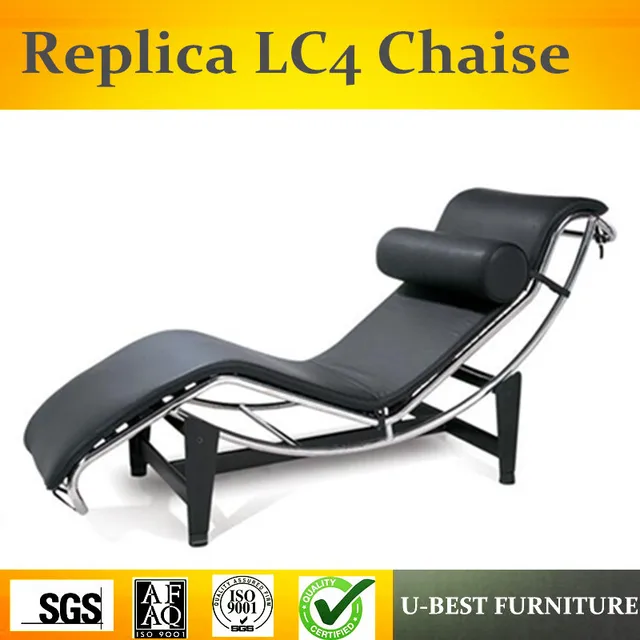The square image prominently features a modern black leather recliner chair named the Replica LC4 Chase. Central to the composition, the chair boasts a sleek design with a black base and a metallic chrome frame, enhancing its sophisticated appearance. The chair's ergonomic structure, complete with a headrest, is designed for comfort, allowing for a relaxed lounging experience in a semi-reclined, 45-degree position.

The top of the image is adorned with an orange and yellow rectangular banner displaying the chair's name, Replica LC4 Chase, in bold black letters, emphasizing its identity. This banner also provides additional manufacturer information, with the name "U-Best Furniture" prominently positioned on the right. On the left, the banner features four logos that indicate various certifications and approvals: SGS, AFAQ, ISO 9001, and a green check mark for Quality Certified, attesting to the chair's high standards and quality. The overall image evokes a sense of contemporary style and assured craftsmanship, making it an effective advertisement for the U-shaped lounger.